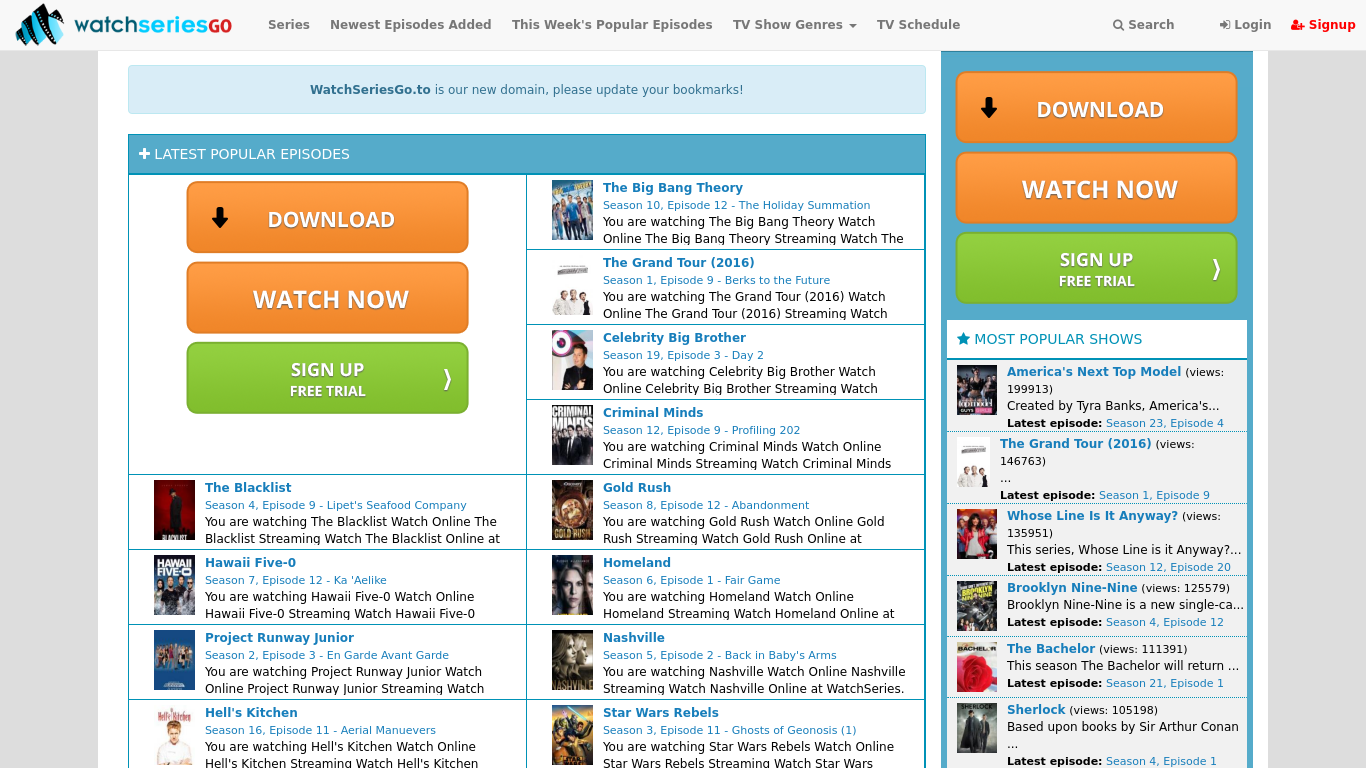This is a detailed caption for the image:

"The screenshot captures a website interface, likely viewed on either a laptop or desktop. At the top of the screen, a very light grey strip extends from left to right, housing the website's logo on the top left. The logo features an old film strip icon in black and light blue, appearing wavy. Adjacent to this, the website name is displayed: 'WATCH SERIES GO,' where 'WATCH' is in small caps grey, 'SERIES' in light blue, and 'GO' in red all caps, forming a single word.

Below the logo, a navigation bar offers several options: 'OPTION SERIES,' 'Newest Episodes Added,' 'THIS WEEK'S POPULAR EPISODES,' 'TV SHOWS AND HONORS,' and 'TV SCHEDULE.' Positioned further right are the 'SEARCH BAR,' 'LOG IN,' and 'SIGN UP,' with 'SIGN UP' highlighted in red.

A blue text box beneath the navigation bar informs users that 'WATCH SERIES GO.2 is our new domain. Please update your bookmarks!' in contrasting light blue background and text.

The main content area showcases a variety of shows users can watch, each with options to 'DOWNLOAD' or 'WATCH NOW,' indicated by orange tabs with 'DOWNLOAD' in white caps and an adjacent black download arrow. Additionally, a light green tab offers a 'SIGN UP FREE TRIAL' with a right-pointing arrow, repeated at the top right of the screen.

Highlighted shows include 'The Blacklist,' 'Hawaii Five-0,' 'Project Runway Junior,' 'Hell's Kitchen,' 'The Big Bang Theory,' 'The Grand Tour 2016,' 'Celebrity Big Brother,' 'Criminal Minds,' 'Gold Rush,' 'Homeland,' 'Nashville,' and 'Star Wars Rebels,' representing the latest popular episodes.

On the far right, a blue star icon precedes the label 'MOST POPULAR SHOWS' in blue all caps. Below this, the featured shows are 'America's Next Top Model,' 'The Grand Tour 2016,' 'Whose Line Is It Anyway?,' 'Brooklyn Nine-Nine,' 'The Bachelor,' and 'Sherlock'.